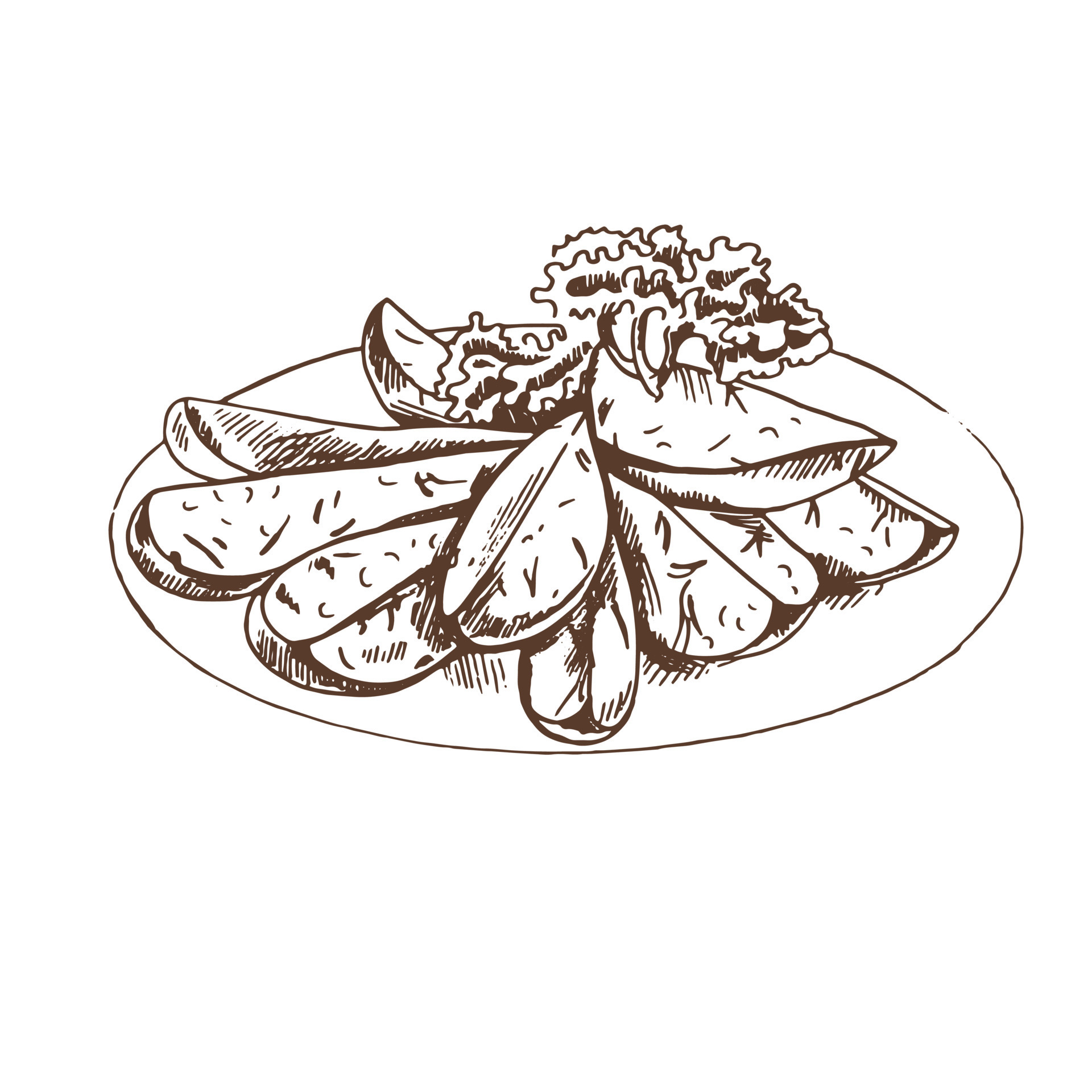This image is a detailed, hand-drawn sketch of a culinary scene presented in a comic book style with a brown-and-white color scheme. At the center of the image is a large white plate with a thin brown outline, slightly cut off on the right side. Resting on the plate are several long slices that appear to be baked potato wedges, each quartered or sixth of a potato, complete with detailed shading lines and sinewy surface texture, including skins on the bottom. The wedges are arranged in a stack, and delicately balanced atop them is a garnish of curly, wavy lettuce leaves, adding a touch of organic complexity. The overall scene is set against an uncluttered white background, bringing focus entirely to the artful arrangement of the potato wedges and their leafy garnish.